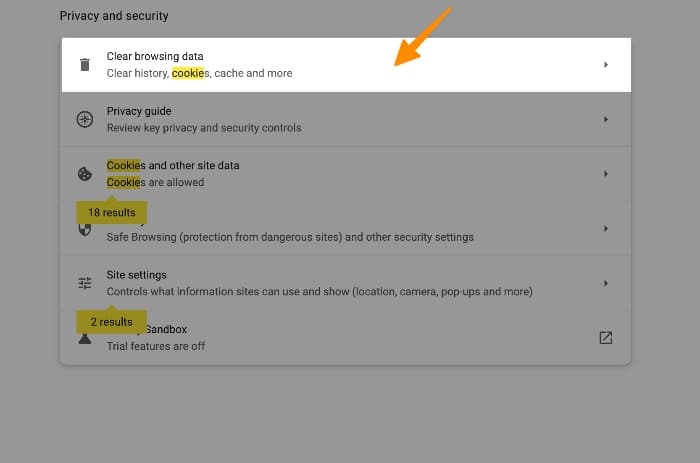This image depicts the "Privacy and Security" settings section within Google Chrome. Key options visible include "Clear browsing data," "Privacy Guide," "Cookies and other site data," "Safe Browsing," "Site Settings," and an entry referring to a sandbox that directs to an external link. An arrow prominently points to the "Clear browsing data" option, likely illustrating a tutorial on how to erase browsing history. In the context of web browsing, the word "cookie" has been searched for and is highlighted multiple times across the page, suggesting an emphasis on managing cookies. Although many menus are collapsed, it is evident from the search results that the word "cookie" appears at least 18 to 20 times on the page. The background of the settings interface is white, with black text for readability. It's noteworthy that selecting the "Clear browsing data" option does not immediately erase data; users must specify the types of data they wish to clear.